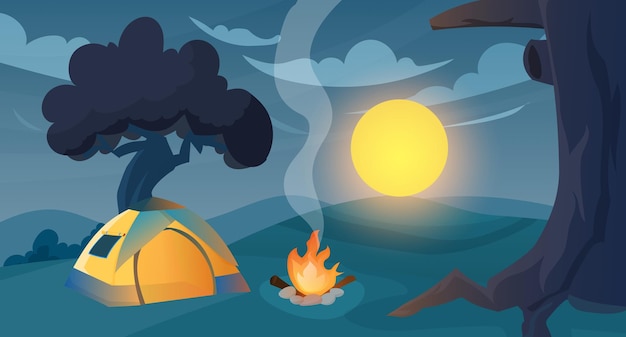This cartoon-style image depicts a simplistic nighttime campsite scene, set against a dark blue sky with pale clouds. A large, luminous yellow moon dominates the background, emitting a soft glow. The scene is set on a grassy area bordered by trees: a barren gray tree stands on the right, while a gray tree with sparse leaves is on the left. At the heart of the image is a small campfire, surrounded by circular gray stones. The fire emits red and yellow flames along with some smoke, and two brown sticks protrude from it. To the left of the campfire, there is a yellow, cone-shaped tent with an open entrance and a small square window. The tent rests beneath the tree on the left, contributing to the cozy, rustic atmosphere of this camping illustration.